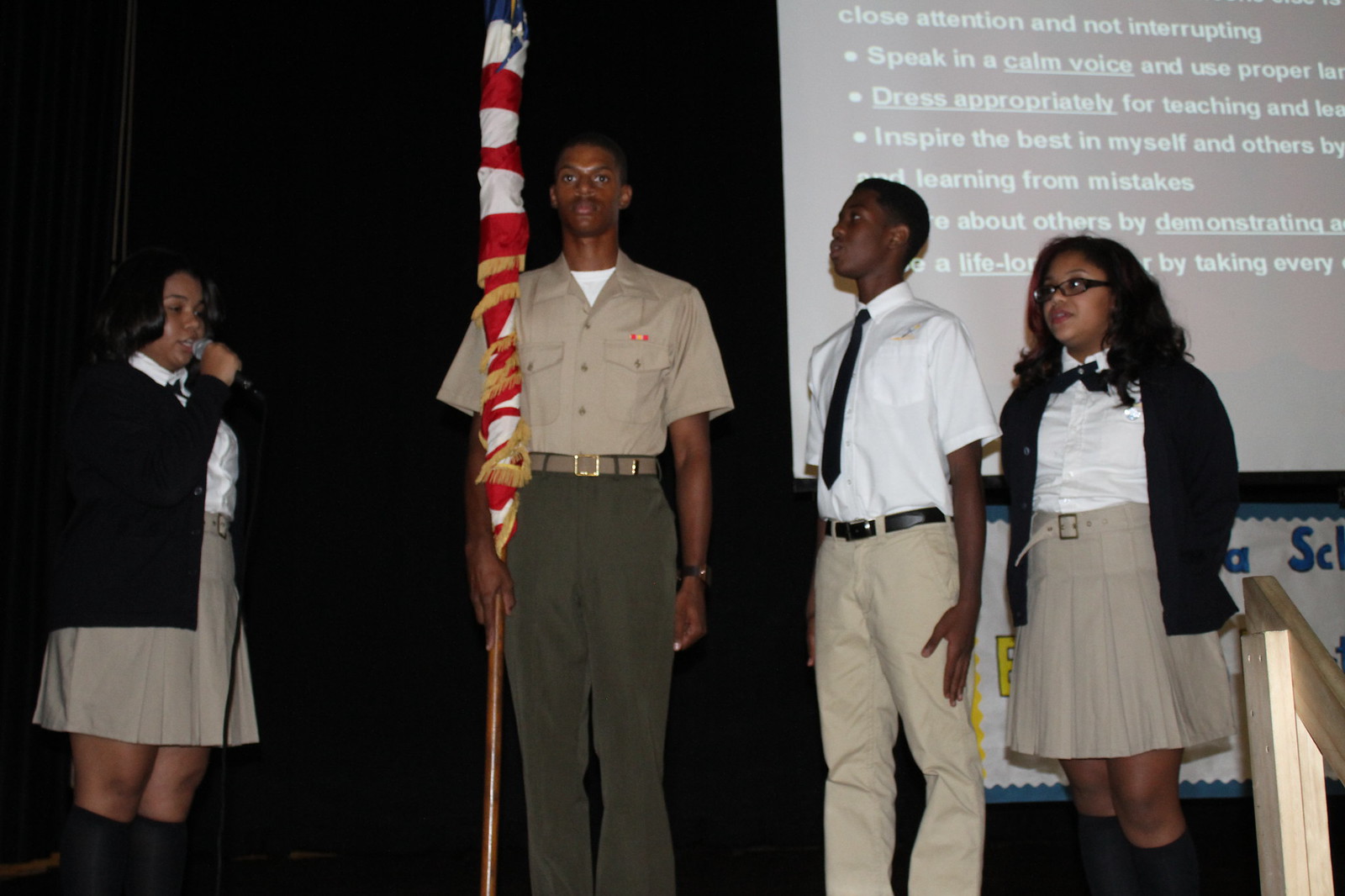This indoor stage photograph features a group of young individuals who appear to be presenting or participating in a formal demonstration. Central in the image stands a young black man, possibly in uniform, wearing a light brown, short-sleeved shirt with pockets, olive-colored trousers, and a light-colored belt in his right hand, alongside an American flag rolled up around a pole. To his right is a younger black boy, dressed in a white button-up shirt with a black tie, and beige pants secured with a black belt; he stands straight while looking toward the person to his left. On the far right and the far left of the stage are two young black women. Both young women wear black jackets over white button-up shirts and knee-length beige skirts with belts. The girl on the left, with shoulder-length black hair, holds a microphone and appears to be speaking while looking right. The girl on the right, who has wavy black hair and wears glasses, looks leftward. Behind them, a screen displays partial text suggesting messages about proper conduct and encouragement, including phrases like "speak in a calm voice," "dress appropriately," and "learning from mistakes." The image conveys a sense of organized participation and educational or instructional purpose.